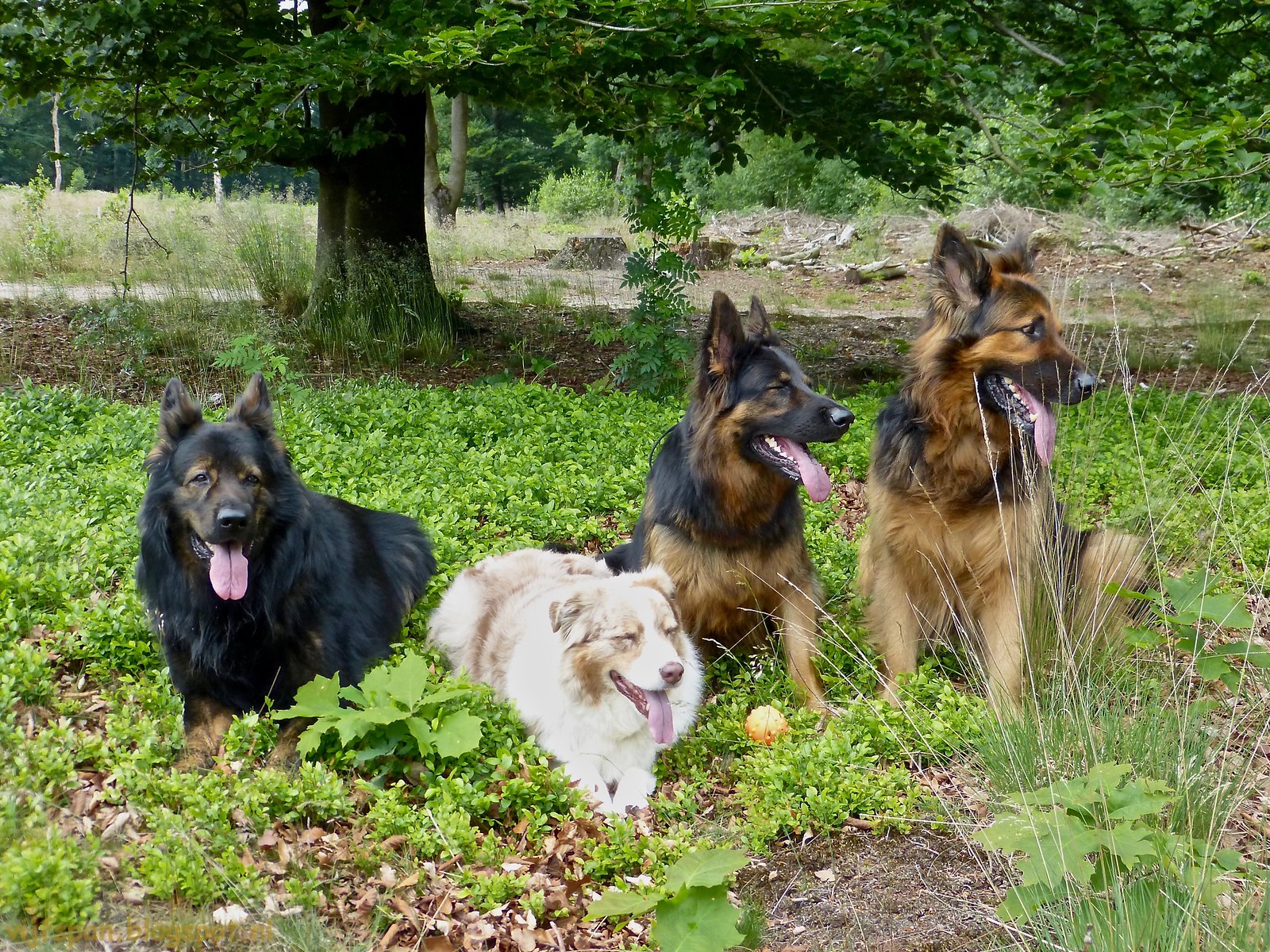This is a photograph taken during a nature walk in a lush, untamed green area. The foreground is teeming with low-growing shrubs and various grasses, contributing to the wild, natural setting. Prominently featured are four beautiful dogs, resting amidst the greenery. Behind them stands a large tree, possibly an oak or cedar, with some climbing vines and more wilderness trailing off into the background, where a pathway is visible.

The dog furthest to the left is very dark, almost black, with a noticeable pink tongue hanging out and looks directly at the camera. Next to this dog is one that appears to be a white and tan Collie mix, with a distinctive brown nose and beige patches. The third dog, seated further right, has the typical sandy coloration of a German Shepherd but with longer hair and some black accents; it also has a pink tongue hanging out. The last dog on the far right is the largest, with long hair and more pronounced sable coloring. All of these dogs seem to have been playing, as suggested by their relaxed, tongue-out demeanor and a yellow ball lying in front of them. The scene captures a serene moment of respite for the canines after what seems to be an energetic play session in the forest.